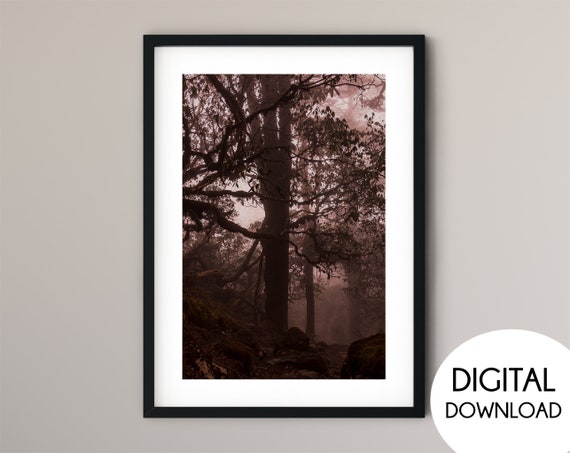This is a photograph displayed as part of an advertisement, housed in a black frame with a white border, mounted on a gray wall. The image within the frame depicts a dark, slightly blurry forest scene shrouded in fog. The photograph primarily features a large tree with a very dark, silhouetted trunk, creating an almost black-and-white effect, though subtle hints of green from leaves and moss can be discerned. The atmosphere is eerie, with branches stretching out like dark, mossy fingers. In the bottom right-hand corner of the image, a white circular bubble contains the text "DIGITAL DOWNLOAD" in large black letters, suggesting the availability of the image for digital purchase.